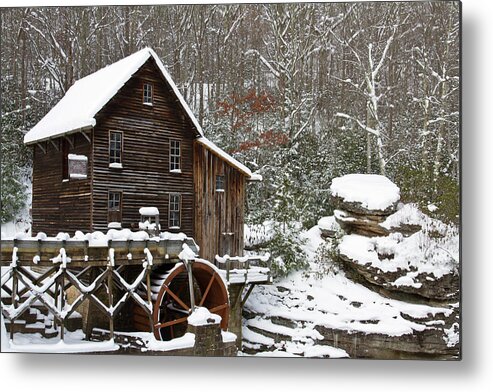The image depicts a serene winter scene outside a rustic log cabin in a bucolic setting. Snow blankets everything—the ground, the roof of the cabin, the branches of the barren trees, and even rocks scattered around the scene. The cabin, likely two stories tall, has four front-facing windows along with a triangular roof. There's an additional triangular section extending from the right side of the house. Prominently in the foreground sits a wooden wheelbarrow with circular, wooden wheels, partially buried in the snow. To the left of the cabin, there is a notable structure featuring a gristmill with a wooden tray on top, laden with snow, suggesting its use for water diversion or grinding. A water wheel is present, its purpose probably related to power generation or irrigation, and intriguing piping extends outwards, also covered in snow. Adjacent stones and possibly a small stream run alongside, with cold but not frozen water meandering through. Barren tree trunks stand behind the cabin, their thin branches accentuating the cold, wintry atmosphere of the entire scene.